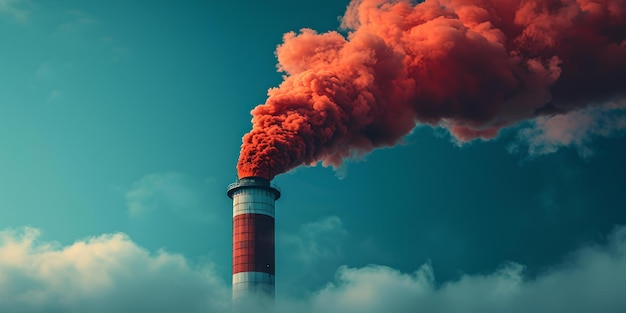This striking rectangular photograph captures a tall, cylindrical smokestack slightly left of center, set against a deep aqua blue sky that darkens towards the top. The smokestack, predominantly white, has a distinctive red band near the top, below which it’s white again, and the very tip appears silver or black. Poking through wispy clouds at its base, the smokestack emits thick, billowing smoke that ranges from a rusty red to orange, casting an ominous contrast against the serene sky. The dense smoke twists dramatically to the upper right corner of the image, almost resembling cotton candy in its thick, voluminous appearance. The overall scene lacks any text or timestamps, solely focusing on the stark industrial element amidst a beautiful yet ironically contrasting natural backdrop.